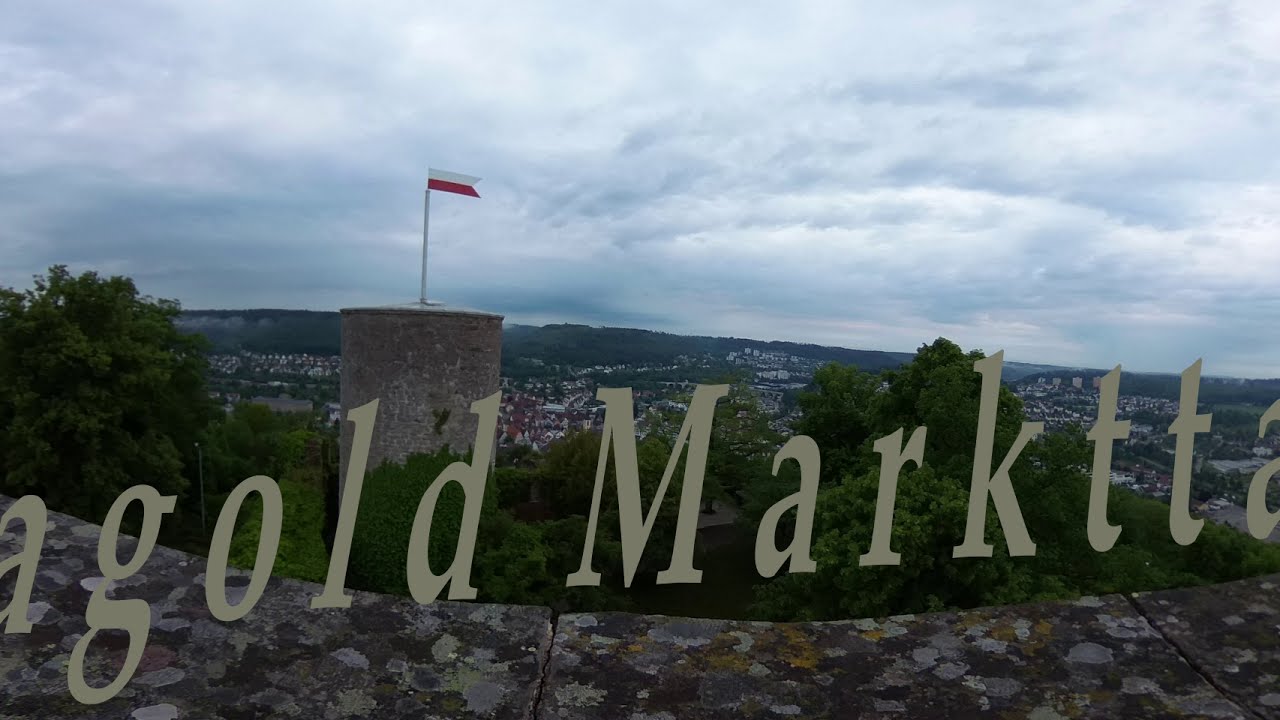The image captures an outdoor daytime scene featuring a complex visual narrative. In the foreground, there's a concrete block with patches of pink, white, and orange paint, suggesting an artistic touch. Upon this concrete surface, individual light gray letters spell out "A-G-O-L-D M-A-R-K-T-T-A" from left to right. The surface appears to have two distinct dividing lines, one just left of center and another in the right corner. Directly behind this ledge, a row of densely packed dark green trees filled with leaves is visible.

To the left of the frame stands a cylindrical brick structure with a flagpole, displaying a flag that's white on top and red on the bottom. This building, likely part of a castle, overlooks a steep drop-off that cascades into the city below. The city is a vibrant mix of colors with buildings topped with red roofs and various architectural styles spread across a hillside.

Further in the distance, rolling mountains stretch from left to right, gently descending. Above, the sky is a collage of cloud formations—some darker on the left, lighter with gray underbellies on the right, and a menacing dark rain cloud in the center. The sky and scenery indicate it is midday, with fluctuating light shining through the clouds, adding depth to the scene. The diverse palette includes shades of gray, tan, brown, yellow, green, white, red, and blue, making for a rich and textured composition.